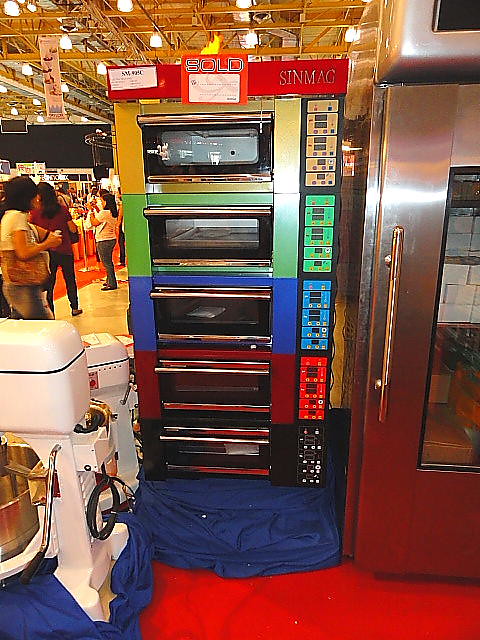The photograph captures a bustling warehouse or store, distinguished by its metal rafters and series of small, illuminated lights overhead. The floor exhibits a striking red hue beneath the various appliances on display. Centered in the image are vividly colored microwave ovens, each adorned with the brand name "Sinmac" and prominently labeled "sold." The ovens are stacked in an array of rainbow hues: yellow, green, blue, red, and black, partially wrapped in blue cloth. To the right of the microwaves stands a sleek industrial freezer with a long horizontal handle and a clear window through which white boxes are visible. Towards the bottom left, a white mixer with a blue stripe and a partially wrapped bowl can be seen. In the background, a crowd of shoppers peruses different appliances and kitchen utensils, accentuating the lively atmosphere of the warehouse.